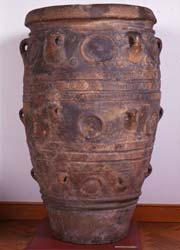The image depicts an antique piece of pottery standing upright on a wood or wood-look tile floor. The pottery is large, cylindrical, and tapers from a narrower base to a wider top. It has a light brown, patinated finish with darker spots and textural indentations, including what might be half-moon shaped designs. The background features a white sheetrock wall with a wood baseboard. There's potentially a handle on the far left of the pot, possibly for carrying it. The photograph is in portrait layout, with the pottery prominently centered against the plain, contrasting background. The setting is devoid of people and text, focusing solely on the detailed and historic nature of the pottery.